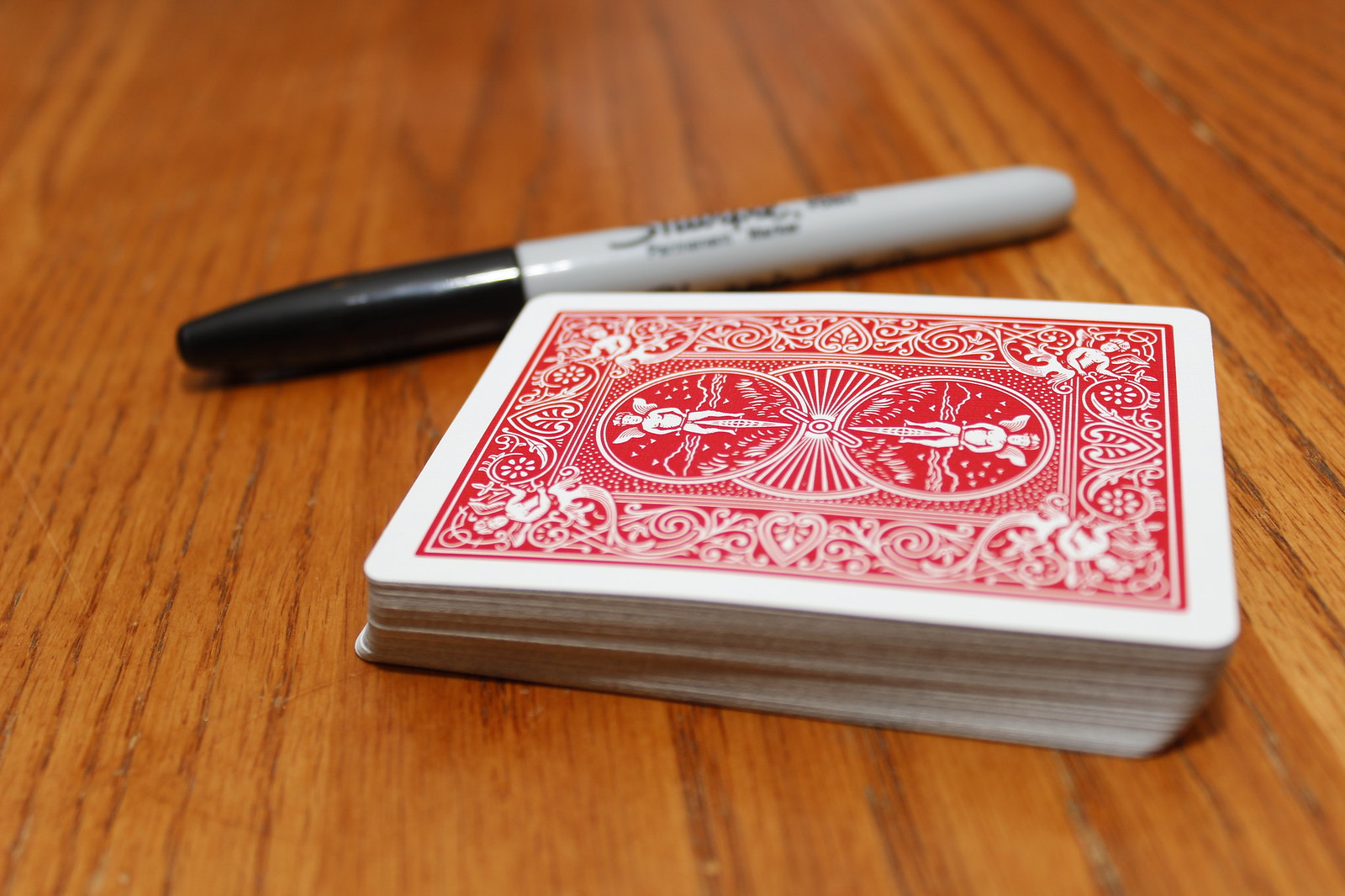A detailed close-up image captures a neatly stacked deck of playing cards resting on a wooden surface. The deck appears complete, its backs adorned with an intricate red and white symmetrical pattern reminiscent of classic Art Nouveau designs. The elaborate motif incorporates curly-Qs, hearts, and elements that evoke the imagery of flowers or perhaps ladybugs.

The wooden surface on which the cards lie is a rich, golden oak hue, suggesting it is either an oak table or an oak floor. Wooden boards with a linear grain run side-by-side beneath the deck, with the grain direction almost but not quite perpendicular to the orientation of the cards. Just beyond the deck of cards, there is a fat black Sharpie marker positioned horizontally.

The photograph provides a near life-size representation, allowing a detailed view of the texture of the wood and the elaborate design on the cards. The overall composition is simple yet rich in detail, highlighting the juxtaposition of the traditional card design against the warm, natural wood grain.